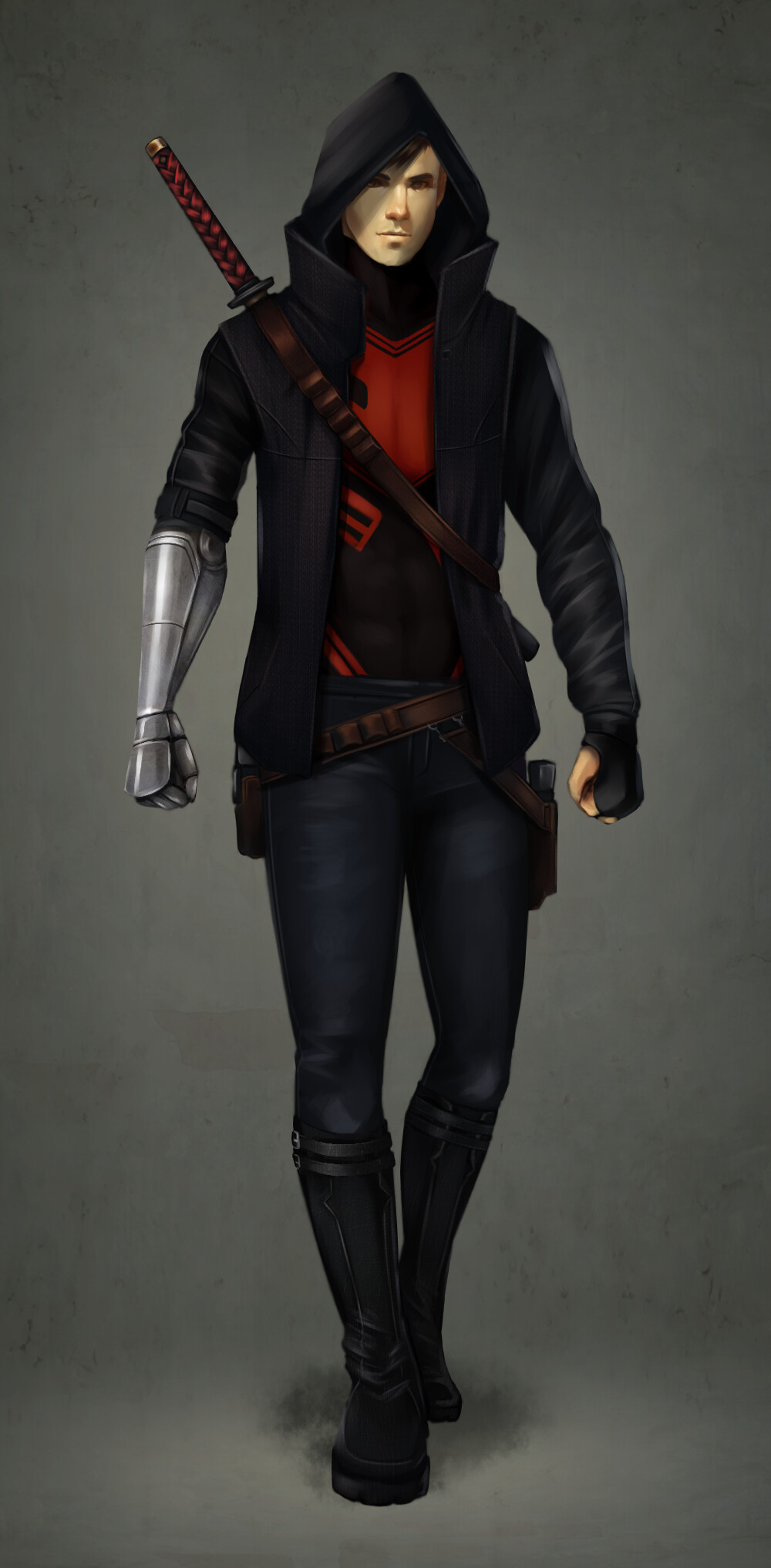This is a highly detailed illustration of a modern, urban ninja warrior, posed like a mannequin displaying a product. The background is a muted gray with a slight green tint, emphasizing the figure in the foreground. The warrior is wearing a black hooded jacket with a high collar, tightly fitted black leather pants, and knee-high black boots. Emanating a mysterious and edgy aura, the individual has emo-styled hair parted to the right, framing a determined face. 

A deep red shirt with black accents peeks out from beneath the jacket, wrapped around the shoulder area. Adding to the intricate ensemble, a fingerless black glove adorns the left hand while a silver, metal armor-type gauntlet covers the right hand up to the elbow, hinting at both style and combat readiness.

A sheath, visible behind the warrior, houses a samurai-style sword, with the hilt pointed over the right shoulder and extending towards the upper left corner. A black belt wraps around the waist, with holsters slung low across the hips, further completing the ninja's tactical and sleek appearance. This comprehensive outfit not only showcases the warrior’s readiness for battle but also lends to a video game-like quality, combining traditional elements with a modern twist.